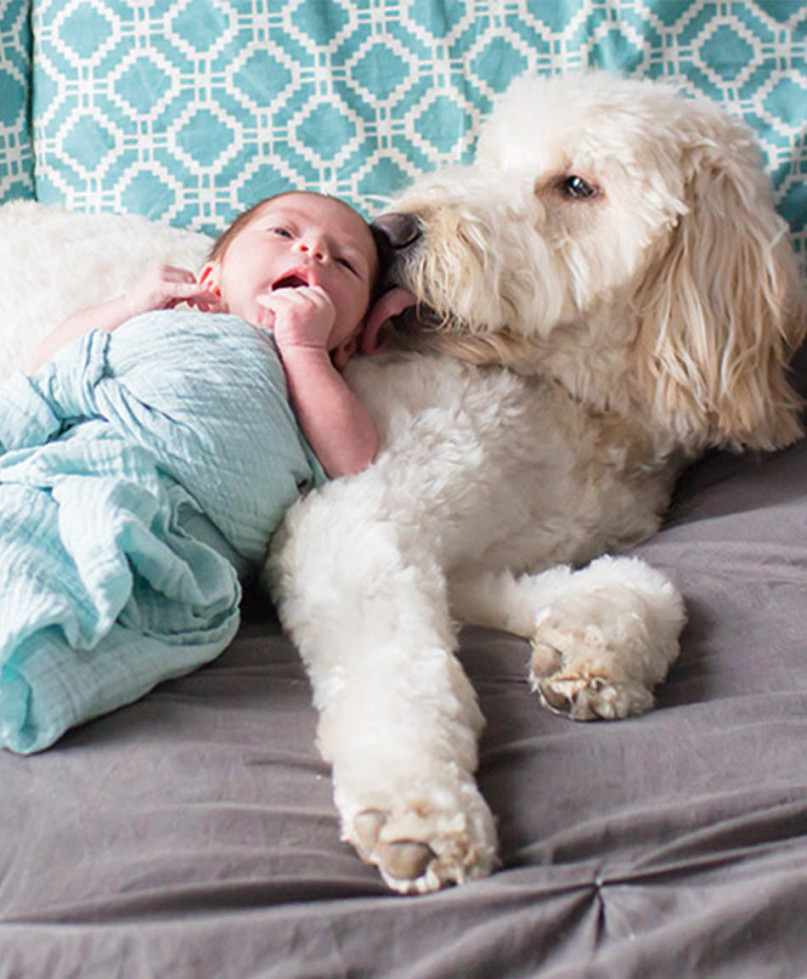This photograph captures a heartwarming moment between a huge, fluffy white dog and an infant. The baby, wrapped in a light blue blanket, lies peacefully on the dog’s chest, both appearing content and serene. The loyal dog, with its soft white fur, is lovingly licking the baby's head and ear. The two are positioned on a gray bedsheet, suggesting they are on a bed or couch. The background features light blue curtains with a white pattern, bathed in sunlight filtering in from a nearby window, adding a gentle, inviting ambiance to the room.